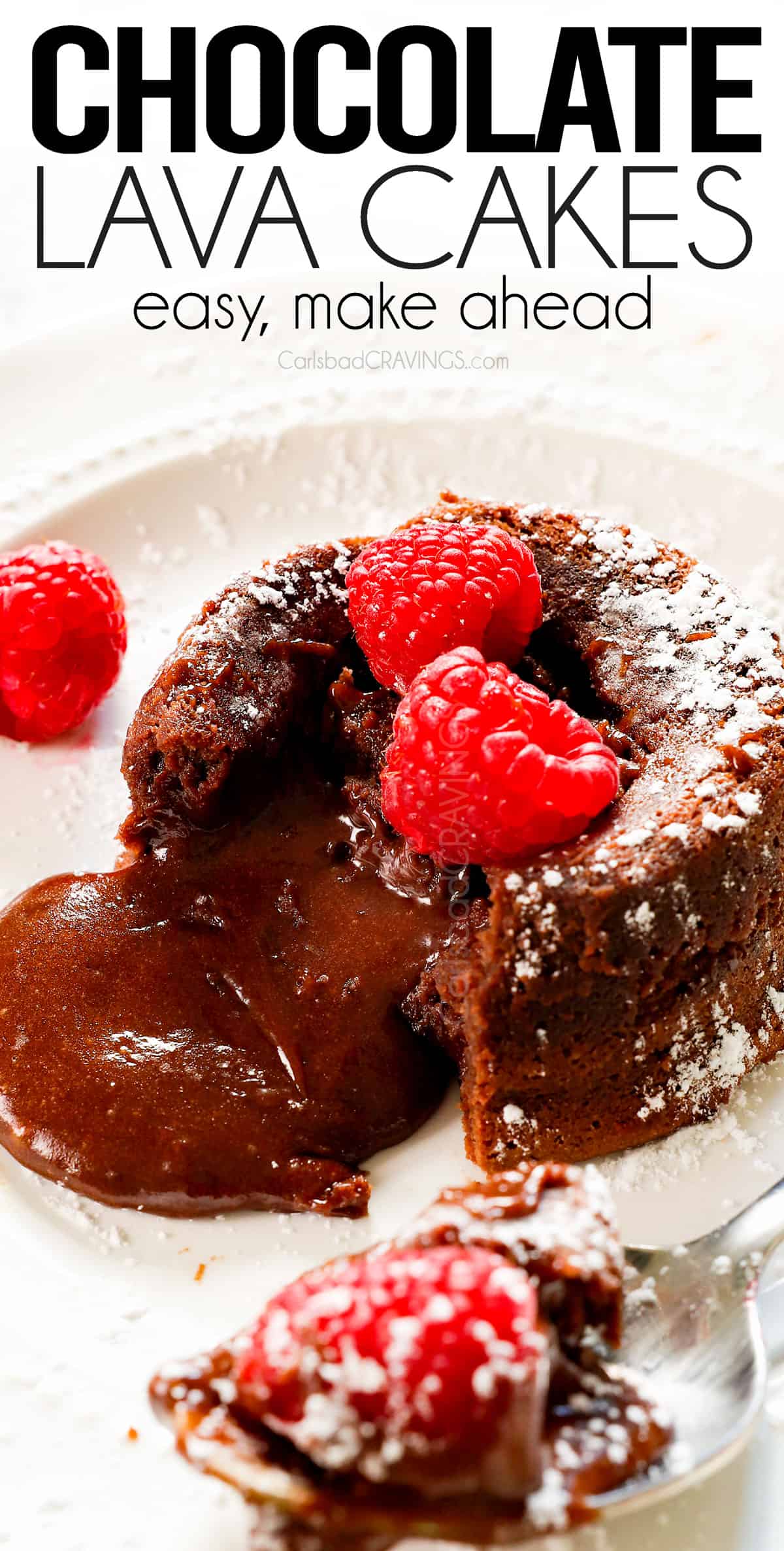This image is an advertisement for a dessert from CarlsbadCravings.com. At the top of the photo, bold, dark capital letters spell out "CHOCOLATE," followed by thinner, black capital letters reading "LAVA CAKES," and underneath, in lowercase thin black letters, "easy, make ahead." Below this text is a mouth-watering chocolate lava cake presented in a white rectangular dish. The brown circular cake has been cut open, revealing rich, dark chocolate fluid spilling out from its center. Two fresh raspberries garnish the top of the cake, with another raspberry positioned to its left. In the foreground, a silver spoon holds a piece of the cake along with a chocolate-covered raspberry. The cake is dusted with powdered sugar, accentuating its rich color, and the entire setup beautifully highlights the decadent, melty core and the inviting presentation of the dessert.